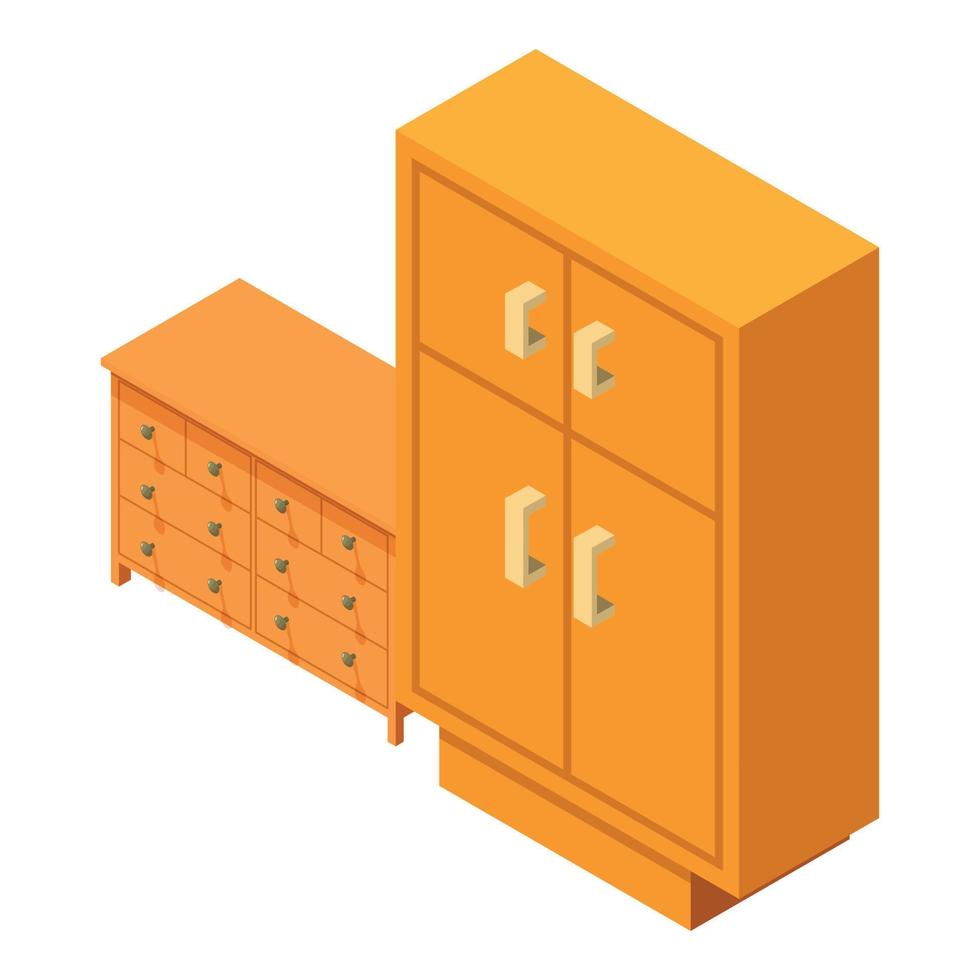The image showcases a detailed digital illustration of two pieces of furniture, prominently displayed against a white background with no text. On the right side of the image is a tall, orange armoire with a square base that doesn't cover its entire bottom. The armoire features two upper and two lower doors, each with metal handles, and is slightly slanted towards the upper left corner, giving it a diagonal perspective. To the left of the armoire stands a similarly colored orange dresser. This dresser, notably smaller in size compared to the armoire, has six drawers, each equipped with metal handles. Both pieces of furniture are designed in an almost cartoon-like style, emphasizing their vibrant orange color and minimalistic lines.